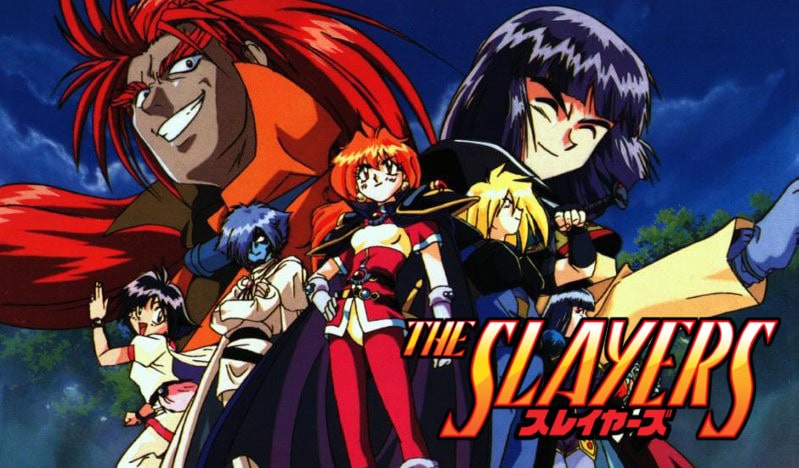In this detailed anime illustration titled "The Slayers," the focus is on a central group of seven characters, rendered in an artful, cartoon style. The background sets a foreboding atmosphere with a dark blue sky peppered with clouds and a misty forest of green trees. The composition is largely centered, with two prominent figures at the top: a large man on the left with a sinister grin, spiky red hair, red bushy eyebrows, and an orange scarf, and to his right, a raven-haired girl with her eyes closed and face scrunched up as she thrusts her right arm forward, clad in a yellow or tan cloak. Below them are five smaller characters: a girl in white with short dark hair, a blue-skinned male with matching hair in white attire, an orange-haired girl in a red outfit, a blonde boy in a blue outfit, and another small girl in a dress with black hair. The anime title, "The Slayers," is displayed prominently in the bottom right corner in yellow capital letters with a red and black outline, accompanied by red Japanese text beneath it. The color palette of the image includes shades of blue, white, gray, red, orange, yellow, pink, and purple, enhancing the vivid and dynamic depiction of these characters.